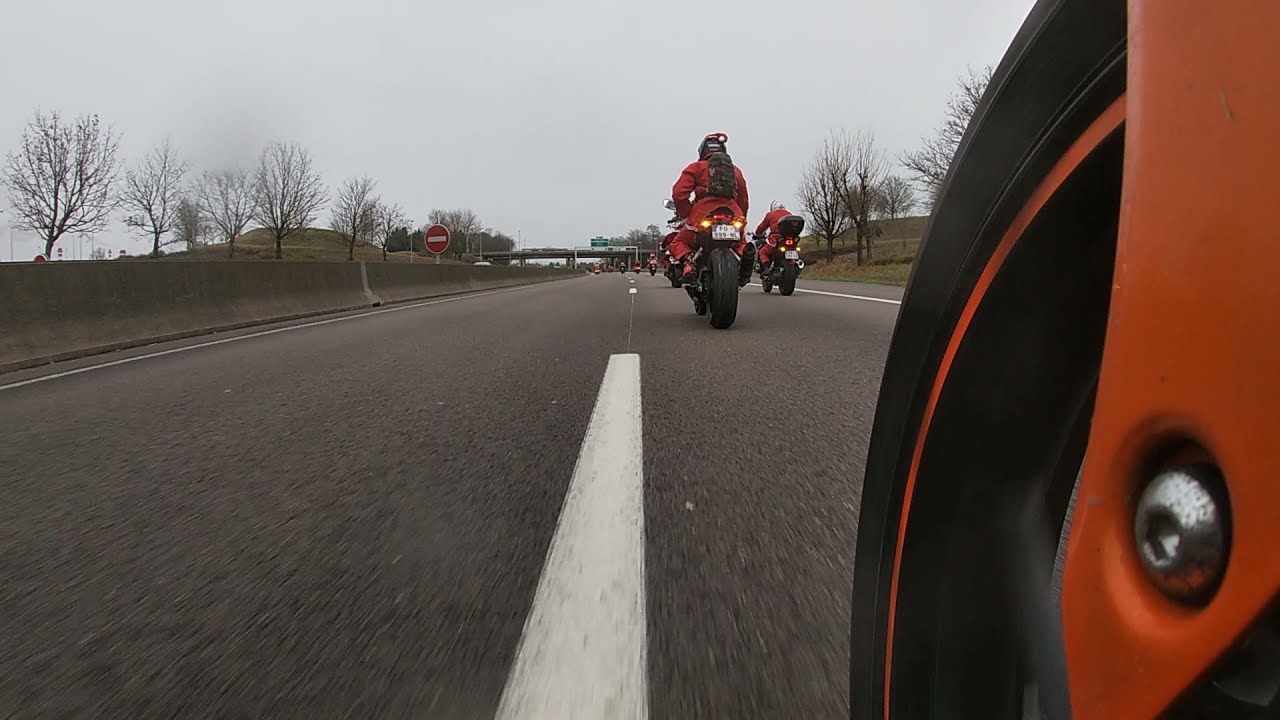The image features a group of motorcyclists riding on a two-lane highway. The riders, dressed uniformly in orange jumpsuits, are wearing either black or white helmets. The photograph captures the scene from a low angle, providing a close-up view of a motorcycle's orange body and black tire on the right side of the image. One rider, clearly visible from the back, carries a backpack, while another to his right sports a white helmet. Ahead, several more motorcyclists are visible, though less distinct. 

To the left of the road, a concrete barrier separates the lanes, behind which stands a grassy hill dotted with leafless trees, suggesting a fall or winter setting. An overhead bridge spans the highway in the distance, accompanied by a large green road sign. In the middle of the concrete barrier, a smaller red circular sign is also noticeable. The overall scene emanates motion, indicative of the ongoing ride along this scenic yet desolate stretch of highway.